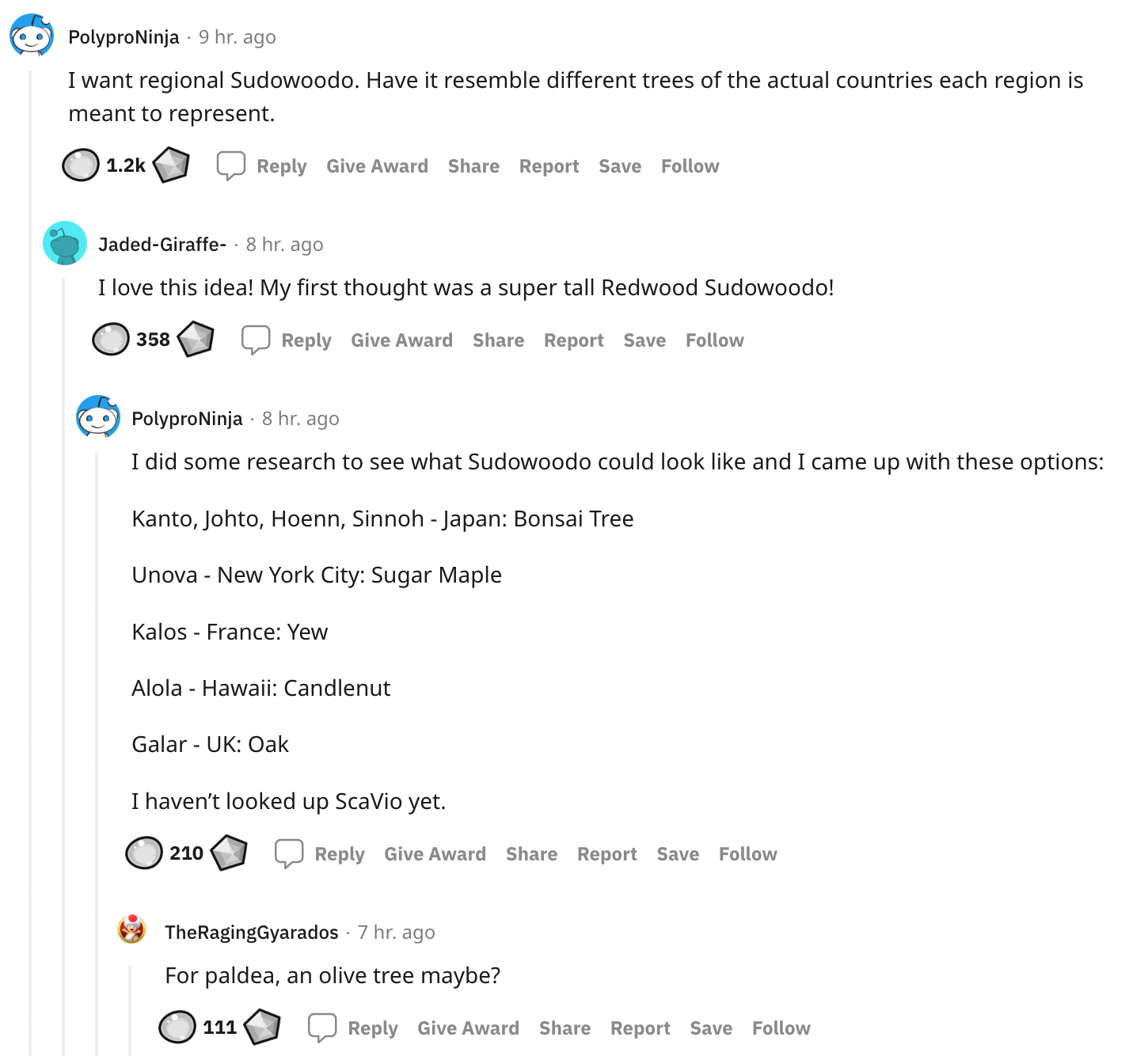This image depicts an online forum discussion about regional variants of the Pokémon Sudowoodo, styled to resemble iconic trees from specific countries. The conversation appears in a comment thread format on a website:

At the top, user Polly Pro Ninja, whose profile is illustrated with a cartoon character, posted nine hours ago: "I want regional Sudowoodo variants that resemble different trees unique to each region's country." Polly Pro Ninja’s statement is supported by a visual of their profile image, which is cartoonish in nature.

Beneath Polly Pro Ninja, user Jaded Giraffe, also represented by a cartoon character profile, replies: "I love this idea. My first thought was a super tall Redwood Sudowoodo."

Polly Pro Ninja then elaborates further with a detailed list: "I did some research to see what Sudowoodo could look like and came up with these options: Kanto, Johto, Hoenn, Sinnoh - Japan: Bonsai Tree; Unova - New York City: Sugar Maple; Kalos - France: Yew; Alola - Hawaii: Candlenut; Galar - UK: Oak. I haven't looked up Scavio yet."

Seven hours ago, Raging Gyarados, another user with a cartoon profile image, contributes to the conversation: "For Paldia, maybe an olive tree?"

Beneath each comment, there's a gray circle with a number to the right, indicating the number of likes or responses. Additionally, a gray diamond-like icon appears below these numbers, likely representing a feature or interaction related to the comments.